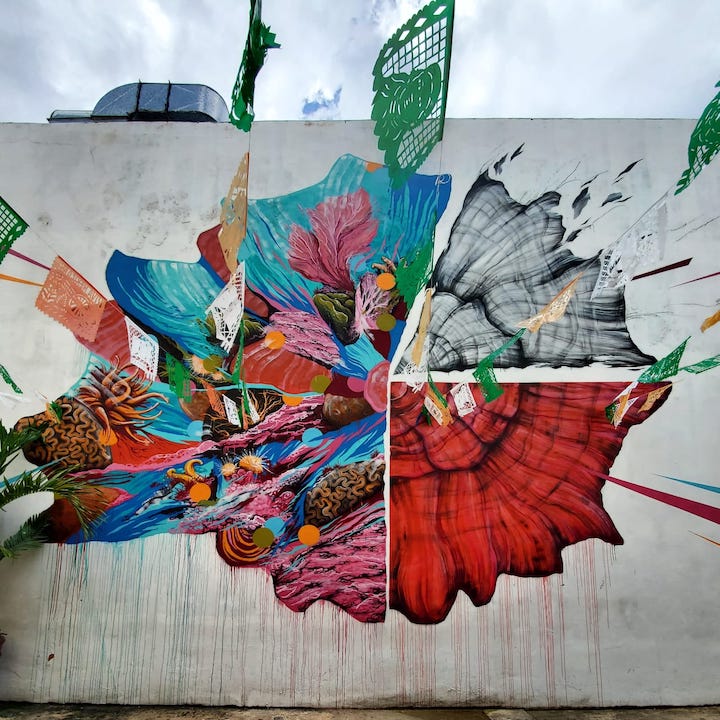The photograph is a square-shaped outdoor image showcasing a graffiti mural on an aged white concrete wall, likely part of a parking garage or similar structure. The mural is divided into three distinct sections, each offering a unique visual experience. The left side depicts an underwater scene with vibrant hues of teal, blue, and turquoise, containing abstract sea life forms like coral reefs, sea urchins, and various ocean plants in shades of pink, blue, and orange. The mural seems to spiral outward, resembling the outer rim of a conch shell. The right side is divided into two segments: the top section is rendered in black and white, while the bottom section features black and red, both illustrating the intricate rings and markings you'd see if a tree trunk were cut in half. The mural shows signs of meticulous detail with paint drips trailing down to the bottom, adding to its dynamic effect. Additionally, small flags in shades of orange, white, green, and a pinkish-beige color hang across the mural, strung up to a point behind the photographer, possibly indicating national representation or celebration.